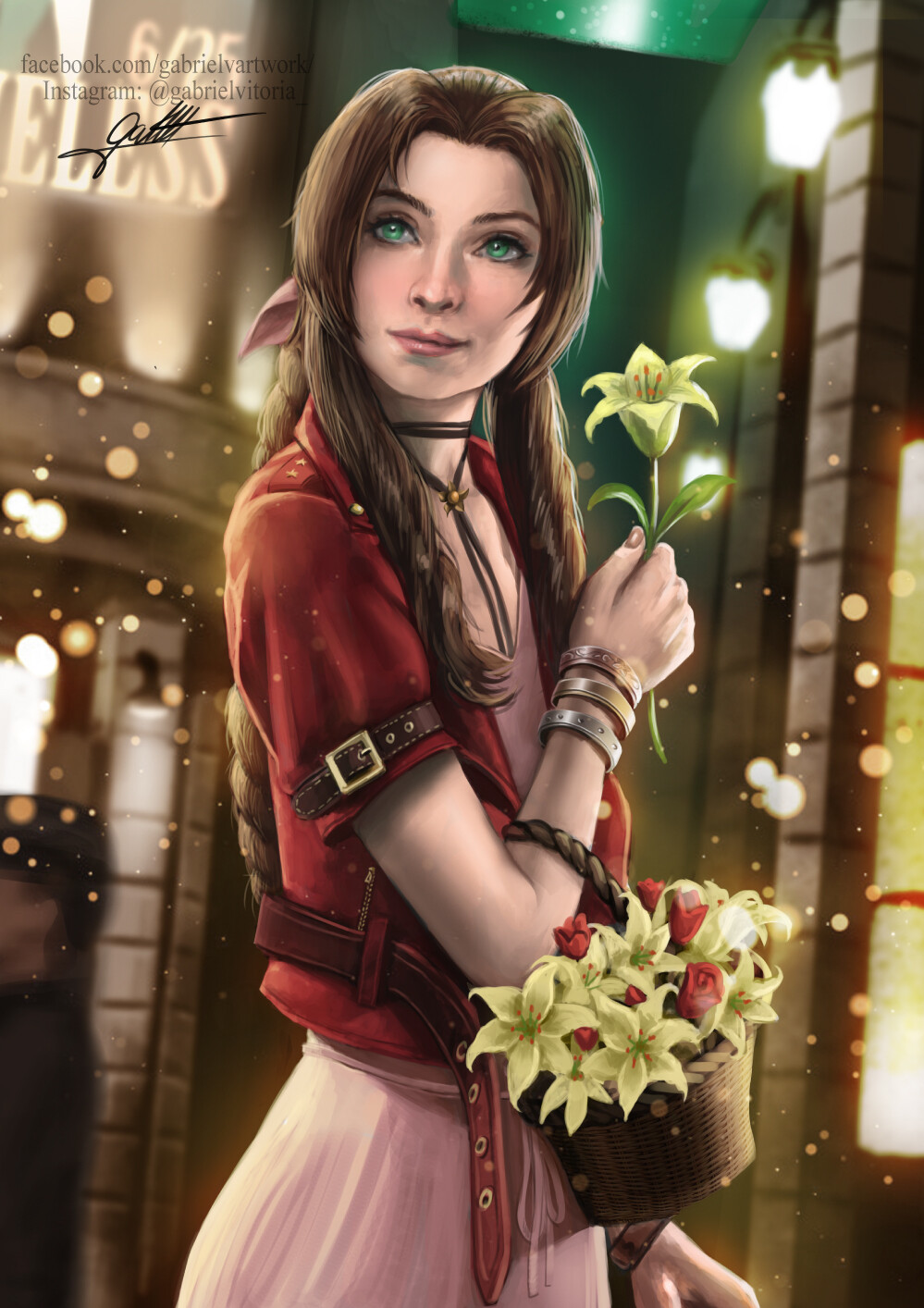The image is a detailed, digital illustration, likely depicting Aerith from Final Fantasy VII, with a city shopping area serving as the backdrop. The scene is set at night, illuminated by scattered lights, suggesting a lively urban environment. The young woman, with fair skin and long brown hair styled in a braid down her back and on either side of her head, faces to her right but looks back to her right, making direct eye contact with the viewer. Her striking bright green eyes are a focal point. She is dressed in a short-sleeved, rust-red jacket adorned with prominent belts over a pink dress. Accessories include multiple bracelets on her right wrist and a necklace. A brown wicker basket, filled with yellowish flowers, red blossoms, green leaves, and possibly white daffodils, is looped over her right arm. She delicately holds one of the yellowish flowers in her right hand. The image is overlaid with faint, gold-colored dots. In the top left corner, the artist's information is displayed: "Facebook.com/Gabrielle V. Artwork" and "Instagram @Gabrielle Vittoria," along with a black signature attributed to Gabrielle Vittoria.